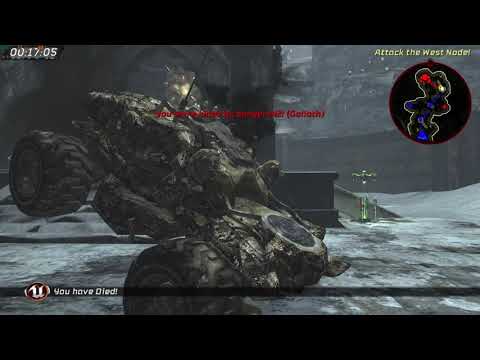The image is a detailed screenshot from a dark, military-themed video game with a snowy and gray environment. Central to the scene is a heavily armored, camouflaged four-wheeled vehicle, resembling a tank or monster truck, that appears to be nose-diving into the ground, its back end lifted and black tires up in the air. The surface below is mostly gray with patches of snow. In the background, there is a stone column or building. The upper left corner of the screen shows a timestamp of "001705" while the upper right corner displays instructions in white text stating, "Attack the West Node," accompanied by a circle containing a stylized map with red and blue areas. The lower left corner contains a black rectangle with red text that reads, "You Have Died," next to a red and white circular logo possibly resembling the letter "U." The overall color theme of the screenshot features various shades of black, gray, and dark brown, with a few touches of gold and red scattered throughout the interface.